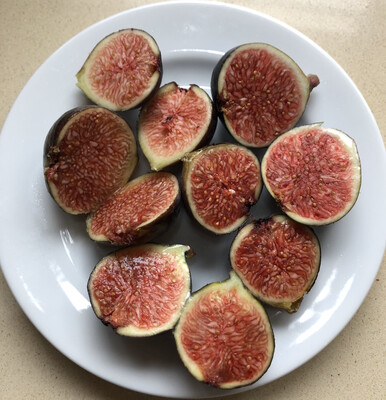In the image, a close-up shot captures a white circular plate occupying 90% of the frame, positioned on an off-white, speckled marble or linoleum tabletop. The plate is slightly cut off at the edges, indicating the zoomed-in perspective. Arranged on the plate are ten fig halves, their interiors facing up towards the camera. These figs display a variety of colors: the skin ranges from a greenish hue to dark, almost black tones, while the exposed flesh is a reddish-maroon interspersed with white pulp. The center of each fig half is densely packed with numerous small seeds that vary in color from yellow to brown. The light source illuminating the scene appears to come from the upper left, casting shadows down and to the right of the fruits. The figs, though slightly dried, reveal intricate patterns in their seeded pulp, enhancing the detailed texture captured in the photograph. The fruits maintain a cohesive arrangement, some leaning against each other, contributing to the organic and textured presentation of this simple, yet striking display.